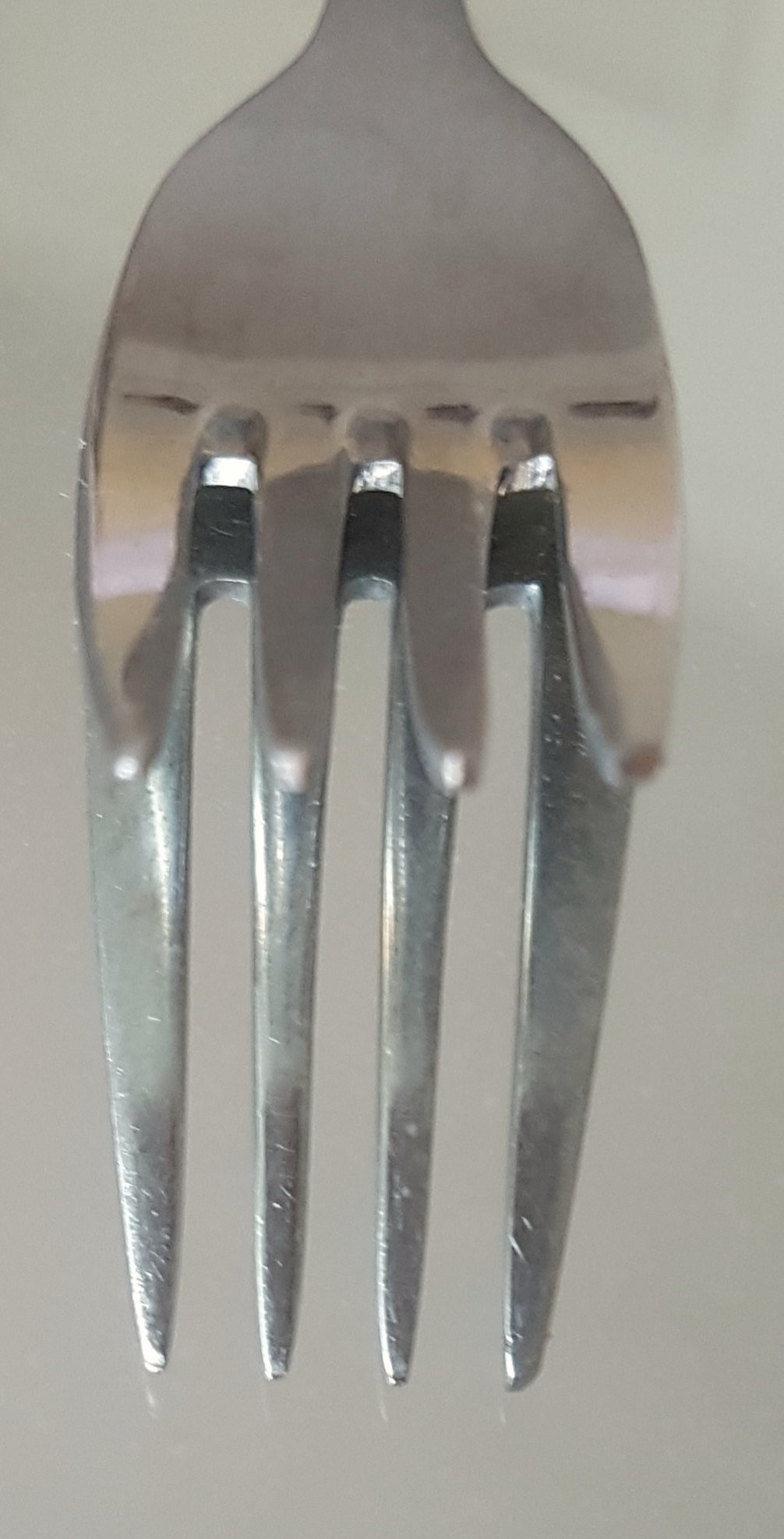The image captures a detailed and close-up view of two stainless steel forks set against a misty, grayish-white background with dark sections. The forks are stacked, with the top fork's prongs pointing directly at the camera. This fork is shiny, silver, and exhibits some pink and white reflections along with a distinctive black line. The bottom fork, which is flipped upside down, has its prongs facing towards the ground and reveals scratch marks and a range of darker silver reflections. Both forks rest upon a reflective surface, allowing the viewer to see the mirrored image of the prongs and the intricate details of their metal surfaces.